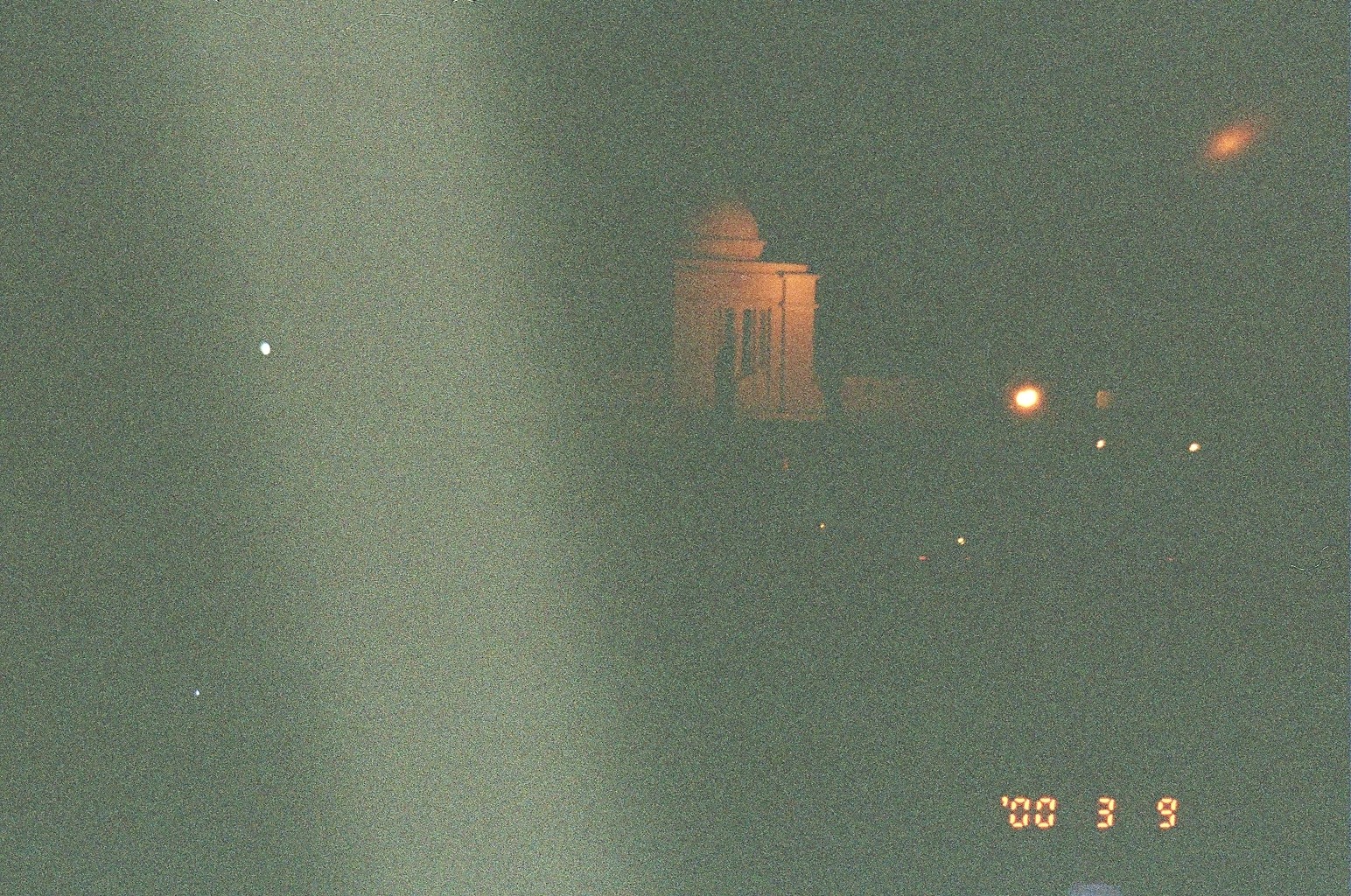This nighttime, grainy photo is significantly out of focus and has a whitewashed, foggy appearance. The image, likely captured by a disposable or security camera, shows a distant, illuminated building reminiscent of those found in Washington, D.C., such as the Lincoln Memorial or the National Mall monuments. The structure features a prominent dome and stone architecture, with possible windows, and is bathed in various lights creating gray, yellow, and white speckled effects. The photo's clarity is poor, with minimal light sources visible, mainly a few orangish lights to the right. There is a time stamp at the lower right corner reading "00 3 9", suggesting it was taken on March 9th, 2000.